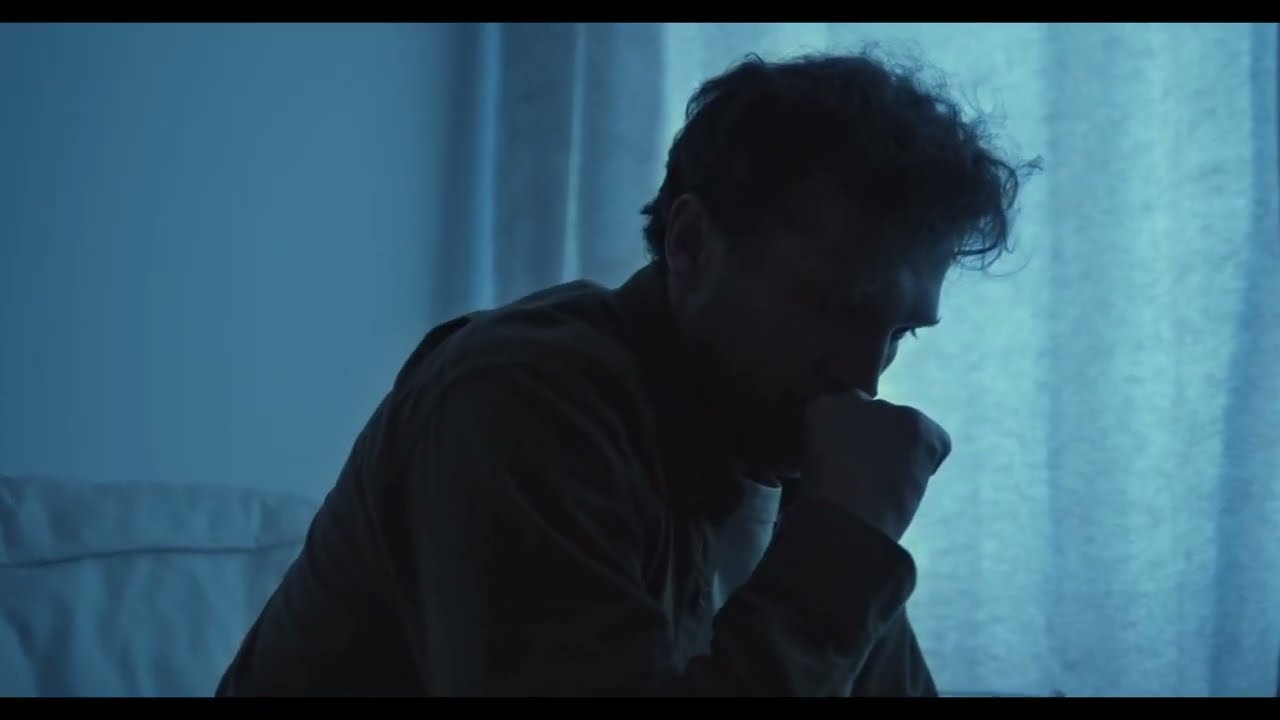The horizontally aligned, rectangular image has a slightly thick black border at the top and bottom, framing a man sitting on a bed in a dimly lit bedroom. The room is bathed in a bluish tint, likely due to a day-for-night shot, casting the scene in shadow and obscuring fine details. The man, appearing forlorn and grief-stricken, leans forward with his elbows on his knees, his right fist pressed against his mouth. His eyes are open but cast downward, suggesting deep contemplation or emotional distress. Partially backlit, his short, messy hair—frizzy and somewhat curly—is highlighted, while his face remains largely obscured. He is dressed in a dark, long-sleeved collared shirt with a hint of a white undershirt visible. The background features a blue-tinted, see-through curtain on the right, allowing faint light to seep through, and a white wall on the left, similarly tinged with blue. A white pillow rests against the wall at the lower left of the image, subtly indicating the presence of a bed.